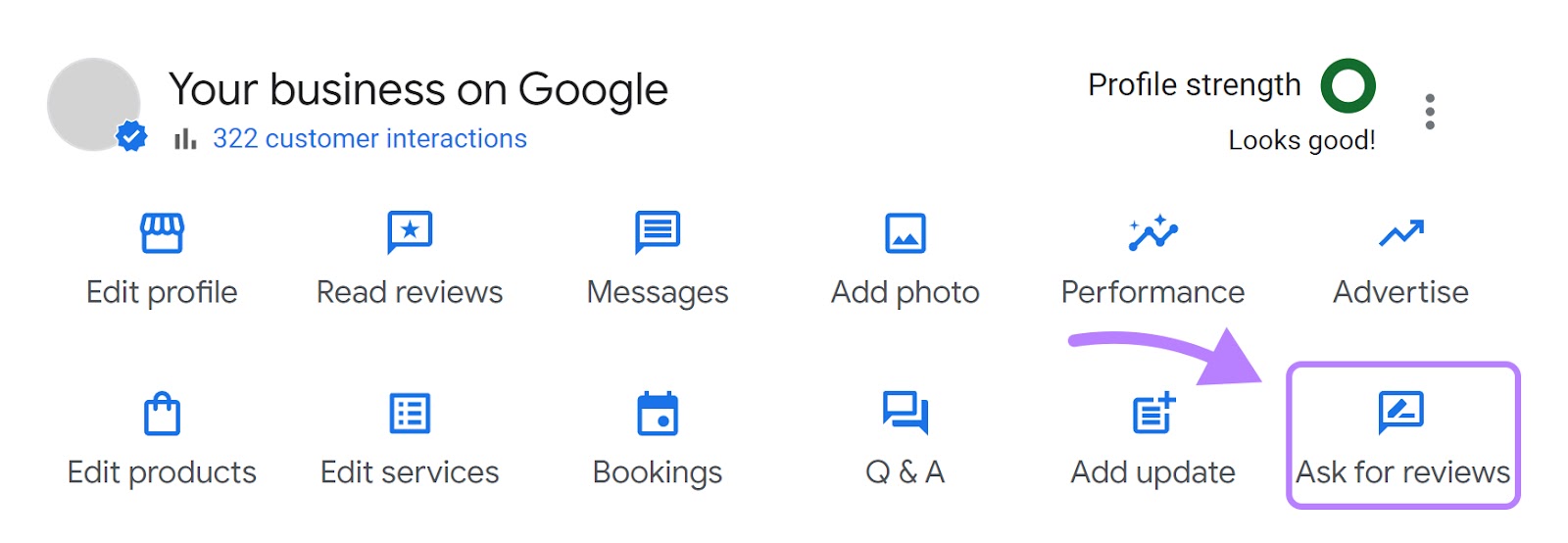This cropped screenshot displays a profile dashboard for Google businesses. In the top left corner, there is a grayed-out profile picture with a blue verified checkmark at the bottom right of the circle. To the right of the profile picture, the text "Your business on Google" is prominently displayed in large black letters. Directly below, the dashboard indicates 322 customer interactions. Further to the right, "Profile Strength" is shown alongside a green circle labeled "Looks Good."

The lower portion of the screenshot features two horizontal rows of six icons each. These icons are blue with their respective names in gray beneath them. The "Ask for reviews" icon, located at the bottom right, stands out with a purple box around it. Additionally, a purple arrow has been edited into the photo, directing attention to the "Ask for reviews" icon and indicating that this is the action to be taken. The careful cropping of the image ensures that users know exactly where to click on the panel.